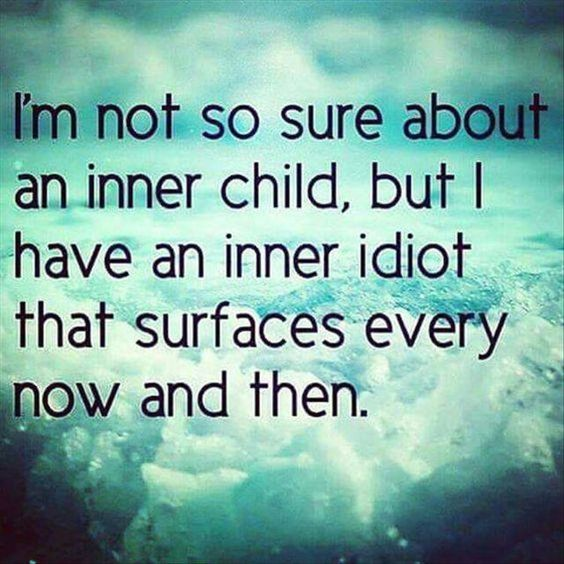A digital image features an intriguing, motivational quote centered against a complex and slightly enigmatic background. The quote, written in bold black text, reads: "I'm not so sure about an inner child but I have an inner idiot that surfaces every now and then." This text is clear and creatively displayed, with the only capital letter being the 'I' at the beginning, and it includes proper punctuation. The background is composed of mountains covered in snow that appear somewhat green-tinted, possibly due to a filtering effect. The snowy mountain scene is blurry, with strong glares from the icy surface adding to the ethereal feel. Dark ice patches are present in both the bottom left and bottom right corners, enhancing the overall dark tone of the image. The colors visible are mostly shades of black, green, white, with hints of tan and light blue, giving the image a unique, slightly surreal aesthetic.